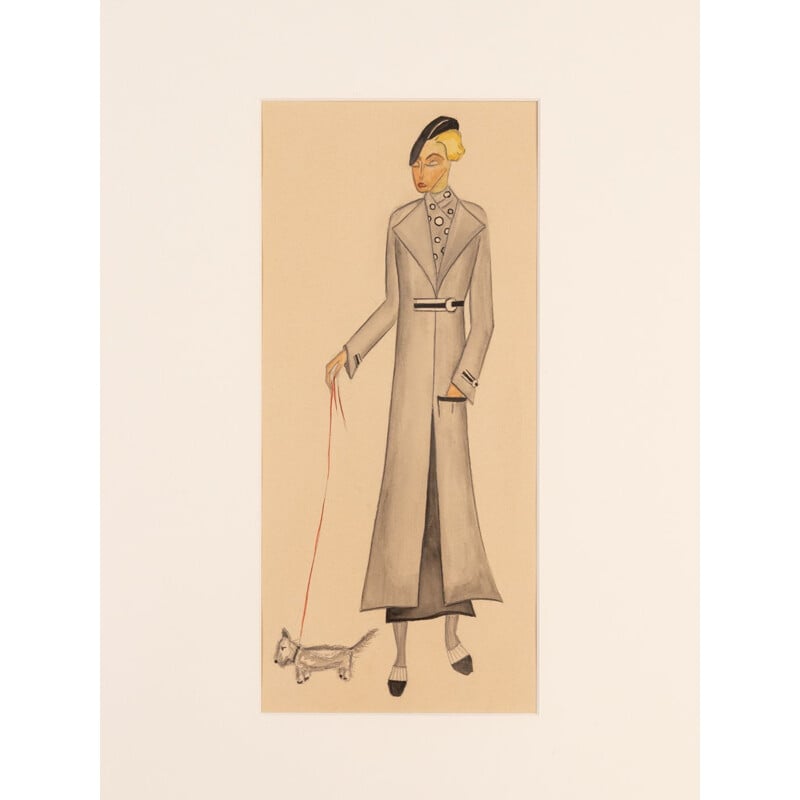This colored pencil sketch, set against a beige rectangular background with a yellowish hue near the edges, features a very tall, elongated woman from a vintage mid-20th-century era walking a small dog. The woman, depicted in a cartoonish and exaggeratedly slender manner, wears a tilted black beret over her short blonde hair. Her facial features include visible eyes, eyebrows, nose, pink lips, and slightly flushed cheeks.

She dons a long, light gray trench coat that extends from her shoulders almost to her ankles. The coat, detailed with a black and silver belt just under her breasts, is open to reveal a darker gray scarf with white polka dots wrapped around her waist, suggesting the appearance of a skirt or dress underneath. Her attire also consists of a long black dress, visible at the coat's opening, and black shoes with white accents.

Her left hand is tucked into her coat pocket, while her right hand holds a red leash leading to a small gray or white terrier at the lower left corner of the sketch. The dog, resembling a Scotty or wiry terrier, stands facing left with its tail pointed backward toward the woman. The entire composition is framed by an off-white backdrop, highlighting the vintage, elongated style of the artwork.